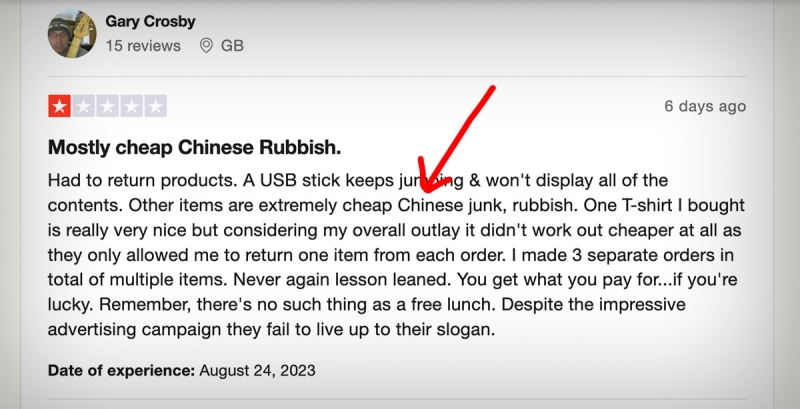This image captures a detailed section of a social media website, featuring a user profile prominently. The profile image, located at the top left, displays a person wearing a hat and glasses, with the neck of a guitar pointing upwards, indicating the user's interest in music. 

To the right of the profile picture, the name "Gary Crosby" is written in bold black text. Beneath Gary's name, it says "Patin Reviews," accompanied by a location icon and the initials "GB," both capitalized. Below this, a horizontal line separates the sections.

Immediately following the separator, a rating system with five stars is displayed, with the first star highlighted in orange, suggesting a low rating. Below the stars, the phrase "Mostly Cheap Chinese Rubbish" is highlighted in black, indicating the review's title.

The main content of the review continues beneath this title. On the right-hand side, you'll notice a timestamp indicating "six days ago." A red arrow points towards a word within the review text, which reads: "Had to return products. The USB sticks keep [blocked by arrow]. It won’t display all the contents. Other items are Extremely Cheap Chinese Rubbish. One t-shirt I bought is really nice. But concerning my overall outlet, it didn't work out cheaper as it [sentence trails off]."

Finally, at the very bottom, the "Date of Experience" is noted as August 24, 2023.